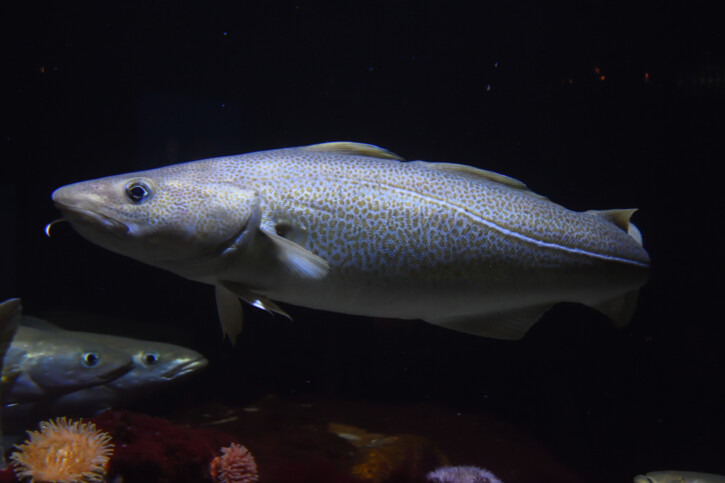This full-color, square photograph captures a vivid underwater scene against an inky black background. Dominating the frame is a large, elongated fish with a pointed snout and a small, antenna-like appendage protruding from its chin. The fish, facing left, features a silver body adorned with brown spots, a white stripe running down its center, and striking black eyes. Its tail curves away from the camera, disappearing out of the frame. In the lower left corner, two smaller fish with silver and gold hues emerge from the scene, also viewed in profile with their black eyes standing out. The bottom of the image showcases four vividly colored plants—yellow, red, purple, and brown—adding bursts of color to the dark, mysterious background. This meticulously detailed composition highlights the intricate beauty of the underwater world.